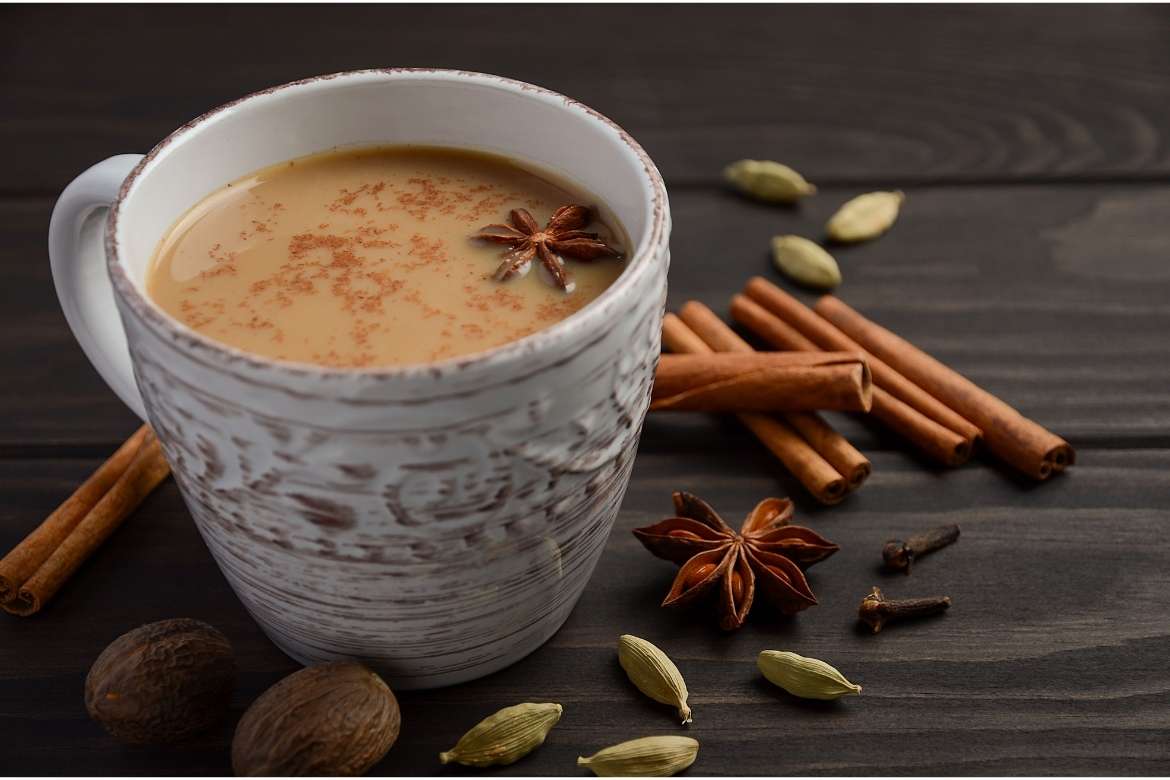This captivating image showcases a white, rustic coffee cup filled with a light tan beverage, likely coffee or tea, sitting on a brown, wood-grain table. The drink appears creamy, with a rich tannish-peach color, indicative of milk or creamer. Floating atop the beverage is an anise star and some grated cinnamon, infusing it with a warm, inviting aroma. Scattered around the mug, which features intricate brown patterns and a homely, textured design, are various spices and nuts: cinnamon sticks, nutmeg seeds, cardamom seeds, cloves, and possibly turmeric. An orange flower adds a touch of vibrant color, enhancing the overall aesthetic. Each item, from the cinnamon sticks' reddish hue to the yellow-brown star anise, contributes to the visually harmonious and fragrant scene, evoking a sense of warmth and coziness. The table's brown wood grain further complements the earthy tones of the spices and the white mug, making this image not just a feast for the eyes, but a sensory journey through smell and taste as well.